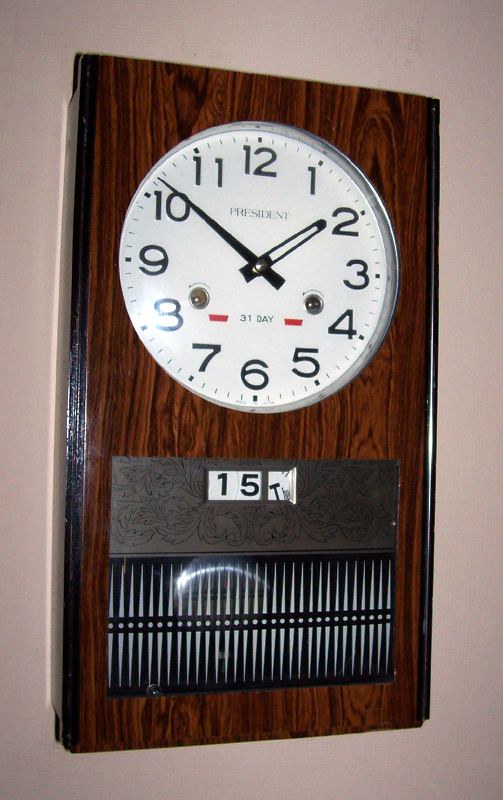The image features a white clock with bold black arrows indicating the hour and minute, prominently displaying the phrase "Present 31 Day" at its center. The clock is mounted on a wooden stump, adding a rustic touch to the scene. Around the clock face, the numbers 12, 1, 2, 3, 4, 5, 6, and 10 are visible, although they appear slightly disorganized, contributing to a bit of convolution. The number 15 is also present, possibly indicating an address. Additionally, the clock face incorporates two red dashes, adding a pop of color to the otherwise monochromatic display. Surrounding the base of the stump are small prickly plants, creating an interesting natural contrast to the manufactured clock.